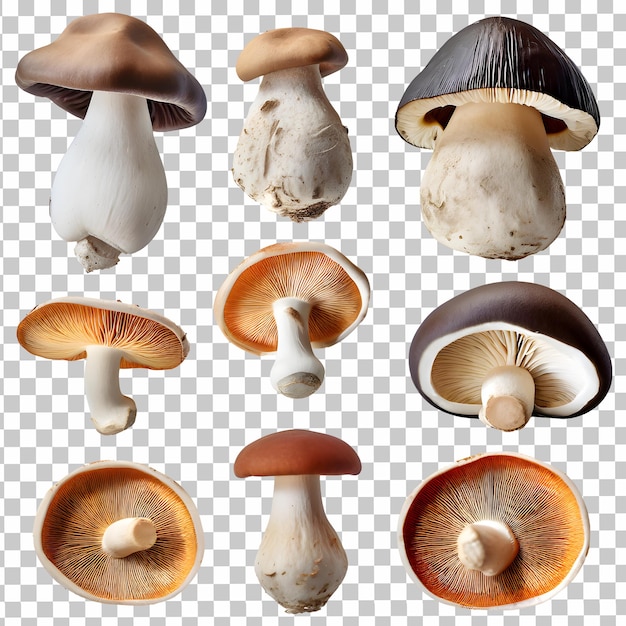This poster features nine distinct mushrooms arranged in a 3x3 grid against a checkered gray and white background, typical of transparent backgrounds in image-editing programs. Each mushroom, showcasing various angles, reveals a diverse range of characteristics. The top row consists of three mushrooms all facing upwards, with the one on the right boasting a thick trunk and a black cap, the middle mushroom sporting a smaller tan head, and the one on the left having a garlic-like bulb with a cowboy hat-shaped top. The middle row has mushrooms tilted to expose their undersides, with dark gills underlined by hues ranging from dark orange to cream tones. Specifically, the middle mushroom in this row is upright, while those on the edges display their undersides completely. The lower row features the bottom left and bottom right mushrooms lying down, revealing their gills, which share a similar dark orange and light brown coloration. There is no text indicating the names or details of the mushrooms, leading to a purely visual exploration of their fascinating differences.